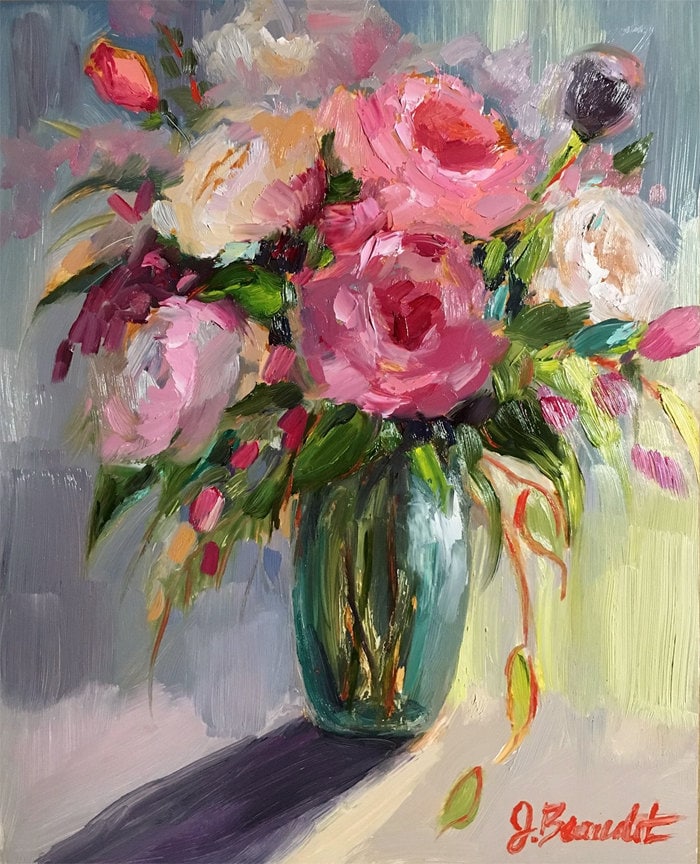The image is a painting, potentially an oil or watercolor, depicting a vibrant arrangement of multicolored roses in a partially translucent blue-green vase. The vase stands against a shaded, multicolored background of grays, yellows, and light blues, casting a distinct dark gray shadow to the left. This background hints at the presence of sunlight with a subtle yellow streak on the table. The bouquet features large, eye-catching roses in shades of light pink, regular pink, hot pink, white, cream, and yellow. Interspersed among the blossoms are unopened buds, especially noticeable on the left, and abundant green leaves that flow outward and downward from the vase. The flowers are supported by brown stems visible through the translucent vase. The painting is signed in cursive with red paint at the bottom right, reading “J. Brand,” though other interpretations suggest it might be “J. Burnett” or similar.